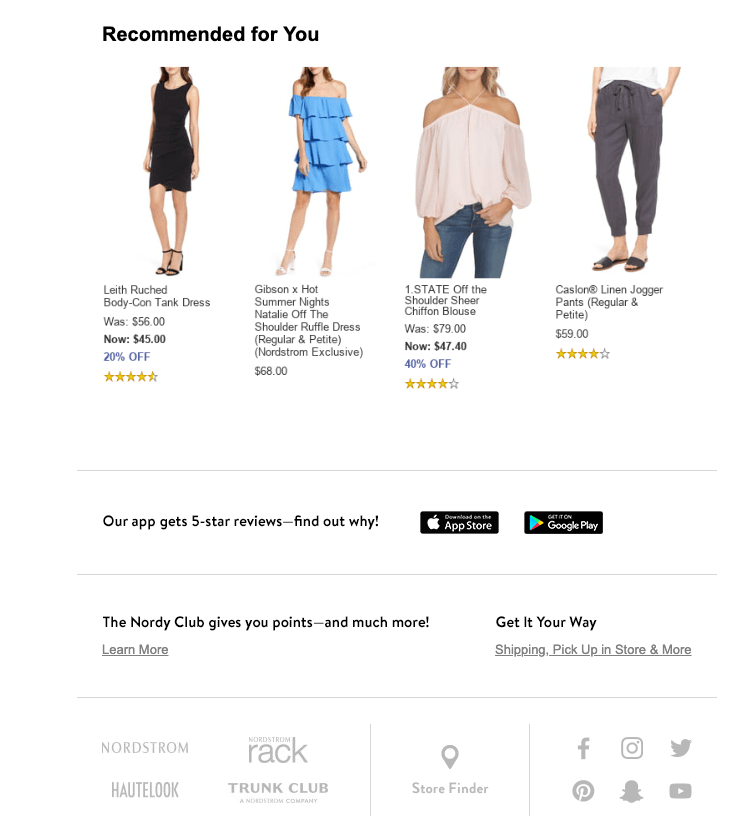The image is a screenshot from a website displaying personalized clothing recommendations. It features four different garments worn by models, each accompanied by a detailed description and pricing information.

1. **Top-Left:** A woman is shown wearing a black dress named "Leaf Ruched Body Con Tank Dress." Originally priced at $56, it is now available for $45, reflecting a 20% discount. The dress has received a rating of four and a half stars.

2. **Top-Right:** This section showcases a bluish off-the-shoulder dress named "Gibson x Hot Summer Nights Natalie Off-The-Shoulder Ruffled Dress," available in both regular and petite sizes. It is exclusive to Nordstrom and is priced at $68.

3. **Bottom-Left:** Displayed here is the "One State Off-The-Shoulder Sheer Chiffon Blouse." Initially priced at $79, it is currently on sale for $47.40, marking a 40% discount. This blouse has received a four-star rating.

4. **Bottom-Right:** The final item is "Cassilon Linen Jogger Pants," available in regular and petite sizes. These pants are priced at $59 and have a four-star rating.

Below these items, there is a section promoting their app, boasting that it receives "four and five-star reviews" and encouraging users to find out why. The advertisement and promotional content continue further down the image.